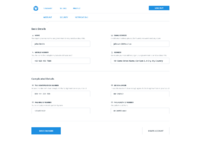The image depicts a blurry and minimized screenshot of a digital interface, making the text illegible. At the very top of the interface, there are three tabs and a prominent blue rectangular button on the right side. To the far left, there's a blue circle. Beneath this top section, there are three additional blue tabs. 

Moving downwards, the information on the screen is organized into two columns. Each column begins with a bold heading, followed by slightly smaller bold subheadings. Below these subheadings, there are text input boxes designated for character entry. Each column contains two such sections, separated by a horizontal line. This structure repeats once more, featuring a heading, subheadings, and text input boxes.

At the bottom of the screen, on the left side, there is a blue button, while on the far right side, there is a white button. The blue buttons, located diagonally at the top right and bottom left of the interface, stand out prominently. The top of the page also features some information written in blue text. The interface does not have any visible borders or distinct endpoints at the bottom, creating an open-ended appearance.